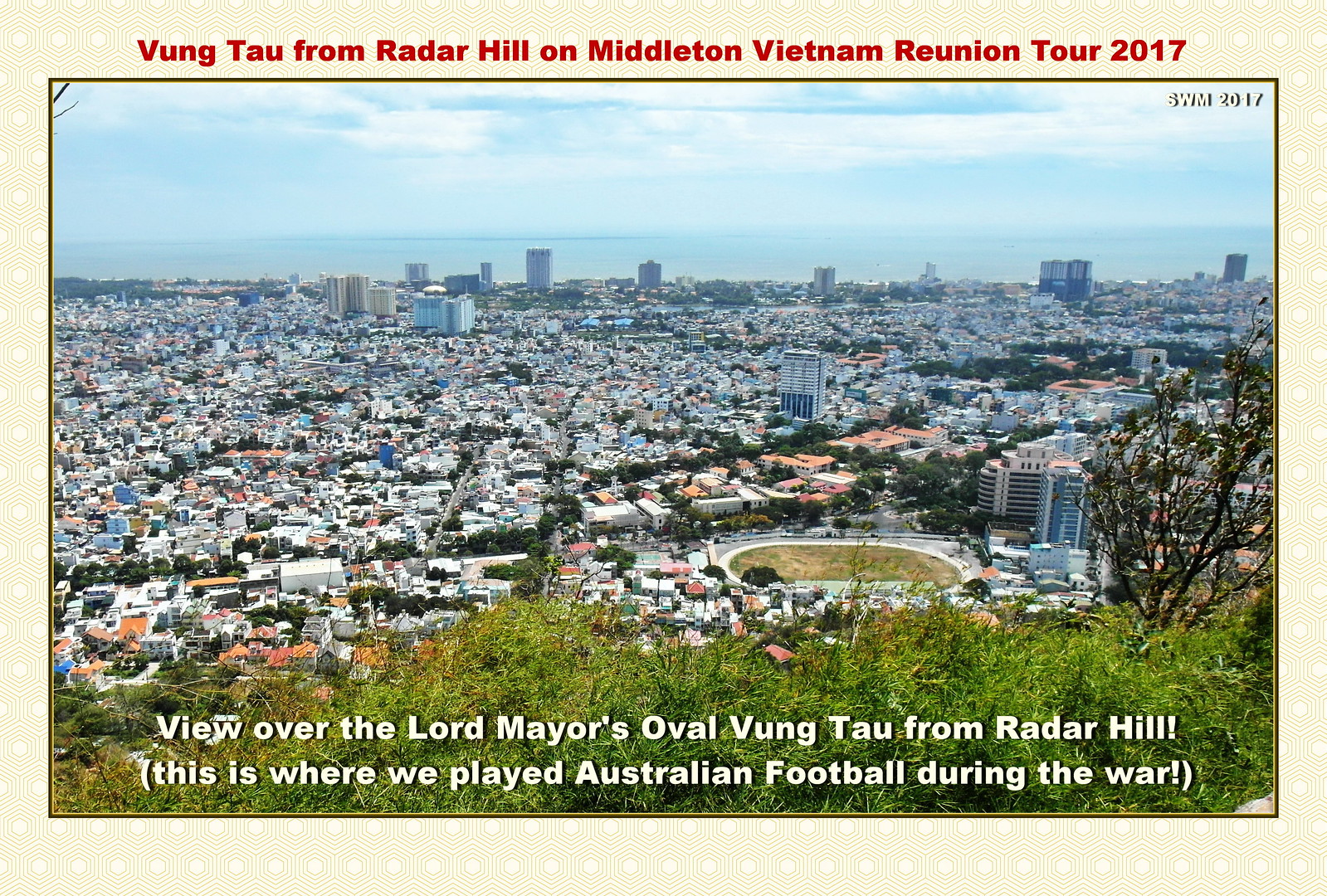The photograph captures a panoramic view of Vung Tau from Radar Hill, taken during the Middleton Vietnam Reunion Tour 2017. At the top, bold red text reads: "Vung Tau from Radar Hill on Middleton Vietnam Reunion Tour 2017." The bottom of the image, superimposed in white text over a grassy foreground with scattered bushes and a small tree on the right, reads: "View over the Lord Mayor's Oval, Vung Tau from Radar Hill. This is where we played Australian football during the war." The center of the image reveals a sprawling cityscape with predominantly low-rise buildings. Towards the right and in the background near the ocean, there are several towering complexes, ranging from 20 to 30 stories. Prominently in the foreground, there is a lush, unkempt field that appears to be a sports field. The city skyline extends towards a massive body of water, likely the ocean, creating a scenic and nostalgic vista.